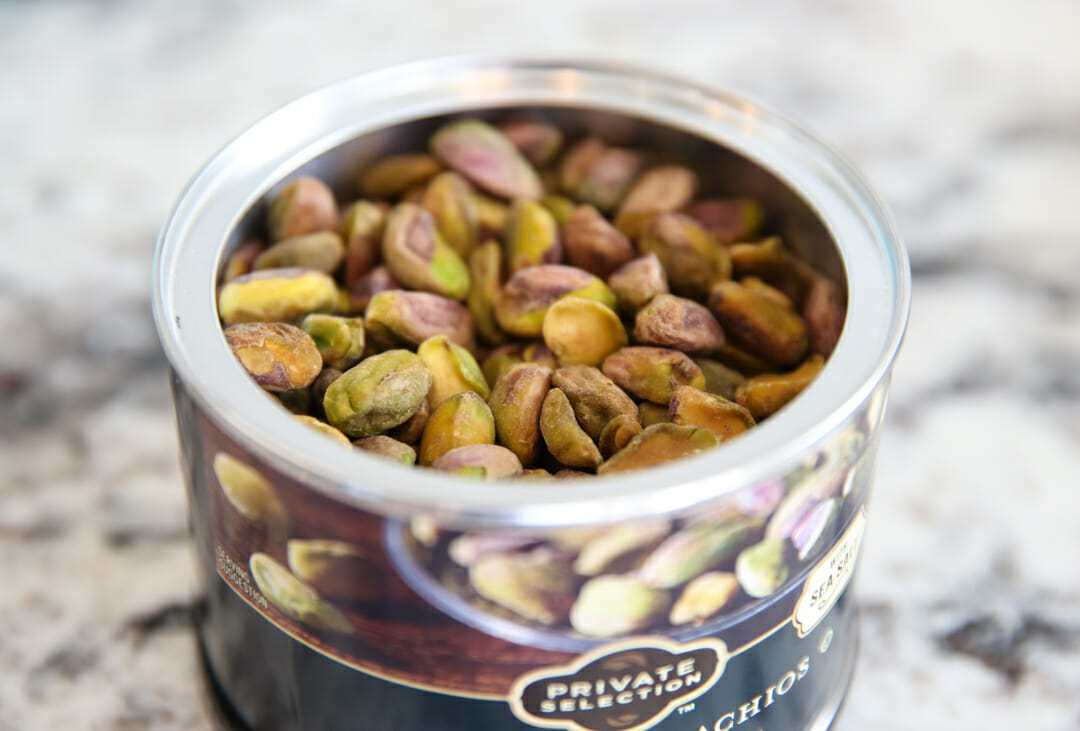The image features an open can of pistachios placed on a white, gray, and black marble countertop. The can is full and does not have a lid, displaying the nuts, which vary in color from medium to dark brown, with some having a greenish hue. The label on the can prominently reads "Private Selection" in white letters within a brown box, accented with light brown leaves at the top and bottom of the text. To the right of this logo, the label also includes the words "Sea Salt" and part of the word "Pistachios." The label is divided into a brown upper section featuring images of pistachios in a bowl and three additional pistachios resting on a wooden table, and a black lower section. The photograph's background is blurry, putting emphasis on the can of nuts.